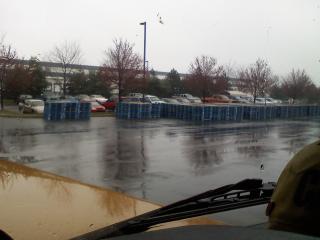The photograph appears to be taken from inside a vehicle, as evidenced by the partial view of the windshield wiper and dashboard. The setting is a parking lot on a rainy day, with the black asphalt appearing wet and reflective. Centered in the image are stacks of blue, square containers, possibly pallets, placed in the middle of the parking area. Beyond these containers, an adjacent parking lot is visible, populated with various cars including a red, silver, and white one. Trees, both green and brown, line the background, some full, others thin or skinny. Additionally, a light post and a large gray and white building can be seen in the far distance, suggesting that the parked cars might belong to individuals visiting or working at this building. The sky is overcast, a uniform light gray with no visible sun or clouds.